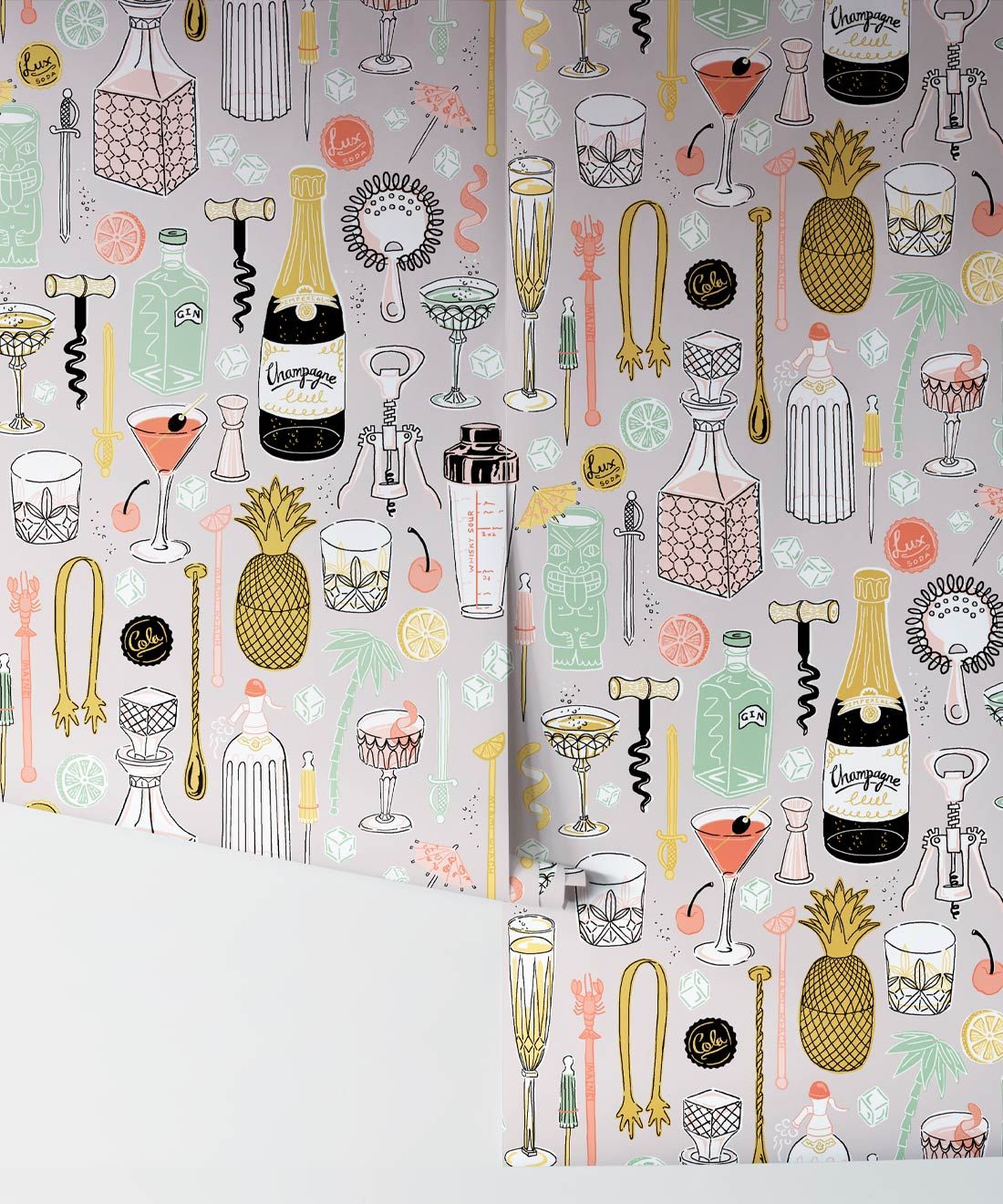The image shows a seamless strip of very stylized, vintage-look wallpaper adorned with a repeating pattern of bartending-themed illustrations on a soft pink background. The wallpaper appears slightly unraveling on the left side, revealing delicate placement details. The design features a variety of items, including vintage champagne bottles, martini glasses, crystal rocks glasses, ornate stirrers, tiki-style glasses, and crystal alcohol decanters. Additional motifs include ice tongs, old-fashioned corkscrews, a small sword or dagger, a can or wine bottle opener, a pineapple, citrus slices, ice cubes, cherries, and palm trees. The color palette consists of gold, blush, silver, and pale blue, giving the wallpaper a charming, almost cartoony and girly aesthetic.